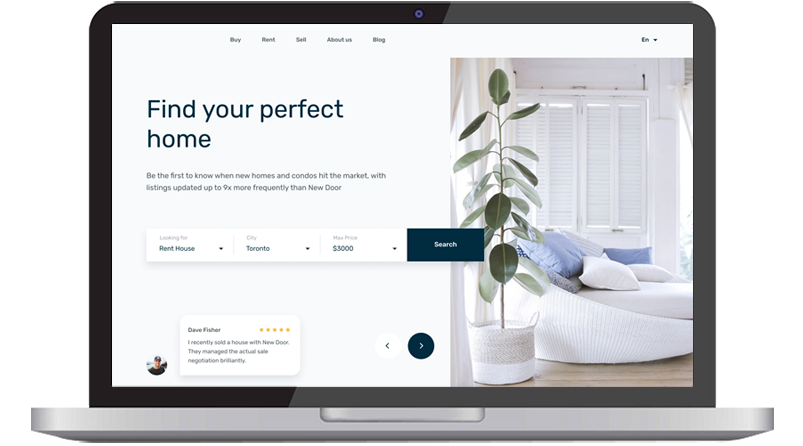The image features a laptop viewed from a straight-on perspective, focusing on its screen. The screen displays a website with a predominantly white background. On the left side of the screen, there is text and options for navigation. A prominent image depicts a serene and modern white living space, adorned with white furniture and distant throw pillows in shades of white, blue, and gray. The room is bathed in natural light from windows covered with white shutters. Dominating the space is a large plant with lush green leaves, almost resembling a small tree, housed in a white pot and standing roughly six feet tall. This greenery provides the main splash of color in an otherwise monochromatic setting. To the left of the image, the website text reads, "Find your perfect home," indicating that this is a real estate platform. The text continues with, "Be the first to know when new homes...," suggesting a feature for staying updated on new property listings. Below this, a panel allows users to refine their search criteria, emphasizing the site's purpose of helping users find their ideal new home.